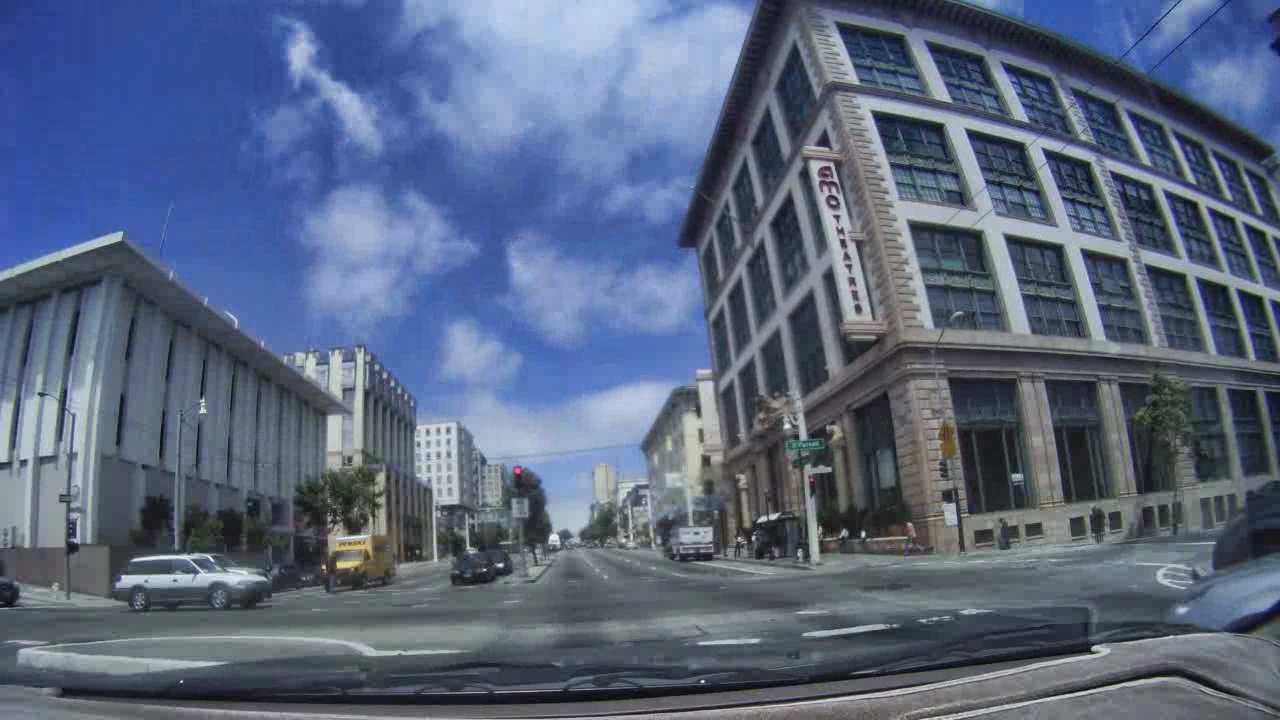The photograph, captured from inside a car, offers a detailed view of a bustling city intersection. Taken through a fisheye lens, the image shows the distorted, wide-angle view from the windshield, revealing a snippet of the dashboard and windshield wipers at the right bottom corner. The sky above features a deep blue with a few scattered white clouds, suggesting it's early in the day. 

Centered ahead is a four-lane road divided by a median strip, with parking on both sides and a red traffic light signaling the car to stop. Across the intersection, a minivan is crossing from left to right, while other cars, including a moving truck, sedans, and SUVs, are waiting at the traffic lights. 

To the right of the intersection is a four-story building adorned with an indistinct sign. On the left, there's a three-story building, and the streets beyond are lined with additional buildings ranging from three to five stories high. This setting, characterized by its office and commercial buildings, reflects a semi-big city atmosphere, possibly near the downtown area but not overly crowded. A green street sign is visible on a metal pole, adding to the structured cityscape of this vibrant urban snapshot.